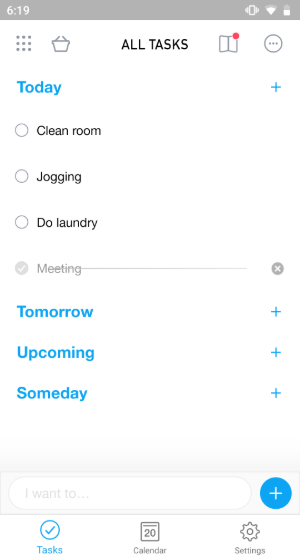This screenshot captures a mobile application interface with a predominantly white background. At the top of the screen, there is a dark gray bar, approximately half an inch in height. On the left side of this bar, the time reads "6:19." Towards the right, several icons are present: a half-full battery icon, a Wi-Fi icon showing three-quarters signal strength, and a phone vibration icon.

Below the time display, within the white background area, a 3x3 grid of dots forms a square pattern. Centered in this section is a shopping basket icon. Adjacent to these icons, in bold black capital letters, the text "ALL TASKS" is displayed. Nearby, a book icon features a small red dot in its top right corner. Further to the right, a circle with ellipses inside has a black border and internal black ellipses on a white background.

On the left, the word "Today" is prominently displayed in bold blue text. Adjacent to this on the right, there is a blue plus sign. Below "Today," several tasks are listed, each with an accompanying icon:

1. A white circle with a black outline next to the text, "Clean Room."
2. A circle icon next to the text, "Jogging."
3. Another circle icon next to the text, "Do Laundry."

In light gray, the task "Meeting" is listed with a line extending across to the right, ending in a gray circle with a black and white X.

Following this section, in bold blue text, the labels "Tomorrow," "Upcoming," and "Someday" are listed sequentially. Each of these labels has a blue plus sign on its right side.

A white search bar runs across the screen with the placeholder text "I want to" in very light gray. To the right of this bar, a blue circle with a white plus icon is displayed.

At the bottom of the screen, several additional icons and texts are visible: a white circle with a blue border and blue checkmark, labelled "Tasks." Next to this, a calendar icon followed by the text "Calendar" in black. Finally, a settings icon with the accompanying text "Settings" in black is positioned on the right.